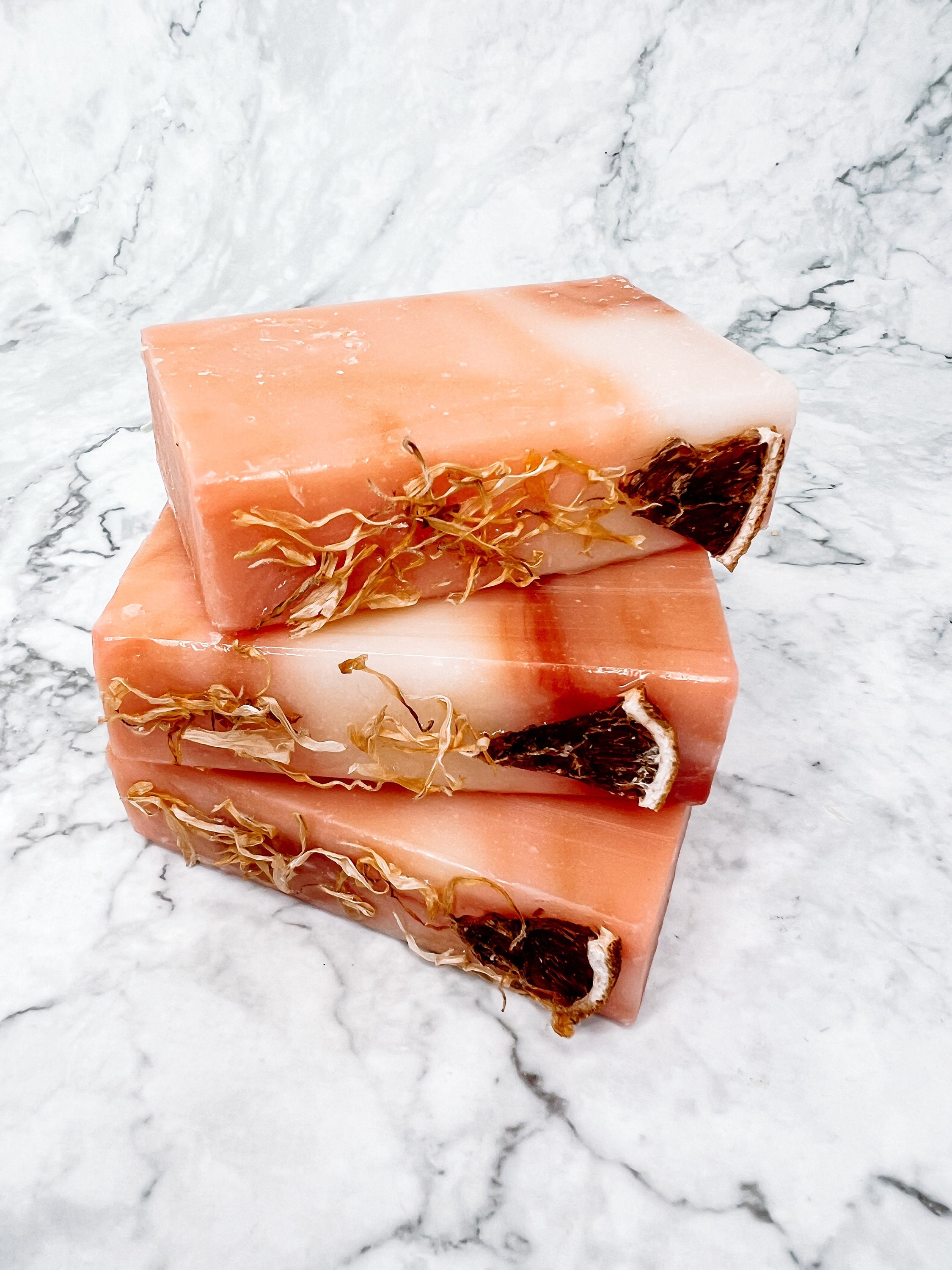The image depicts a close-up of three glossy, peach-colored rectangular slabs stacked on top of each other in a fan arrangement, revealing portions of each slab. Each piece appears to be about an inch thick, three inches wide, and five inches long, and they are set upon a white, black-veined marble countertop. The slabs exhibit smooth, polished surfaces mixed with creamy white and pinkish-orange hues, reminiscent of salmon fillets. Along the sides of each slab, there are thin yellowish filaments resembling straw or hay. To the right of these filaments on each slab, there's a small triangular piece with a white top edge and a brown bottom, which appears sticky and somewhat looks like a garnish or a small pizza slice. The overall appearance suggests a blend of organic and processed elements, visually evocative of polished marble or artisanal soap bars.